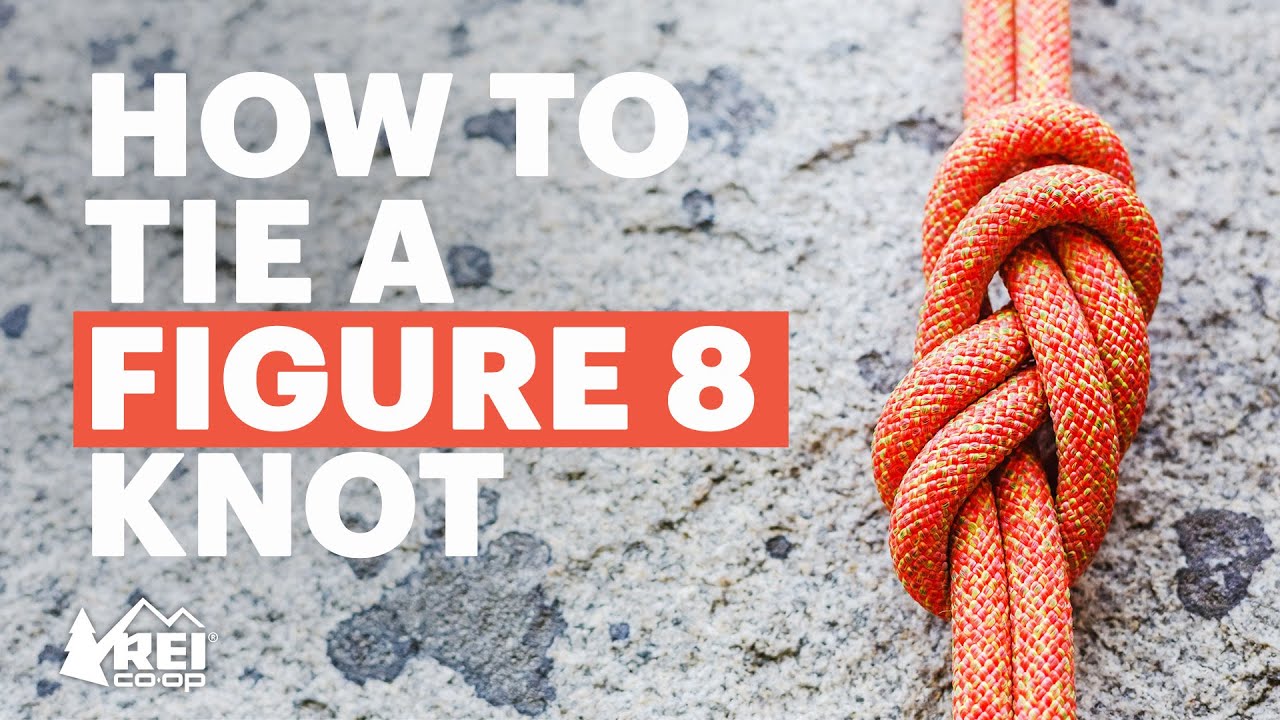The image is a graphic, possibly for a website article from REI Co-op, demonstrating how to tie a figure eight knot. On the left side, large white text reads “How to tie a figure eight knot,” with "figure eight" highlighted by a red border. The background appears to be a rocky surface resembling smooth, finely-grained granite with a few darker mineral splotches. An orange and yellow rope is intricately tied into a figure eight knot on the right side of the photo. At the bottom left corner, the REI Co-op logo is visible in white, featuring a pine tree and a mountain silhouette.